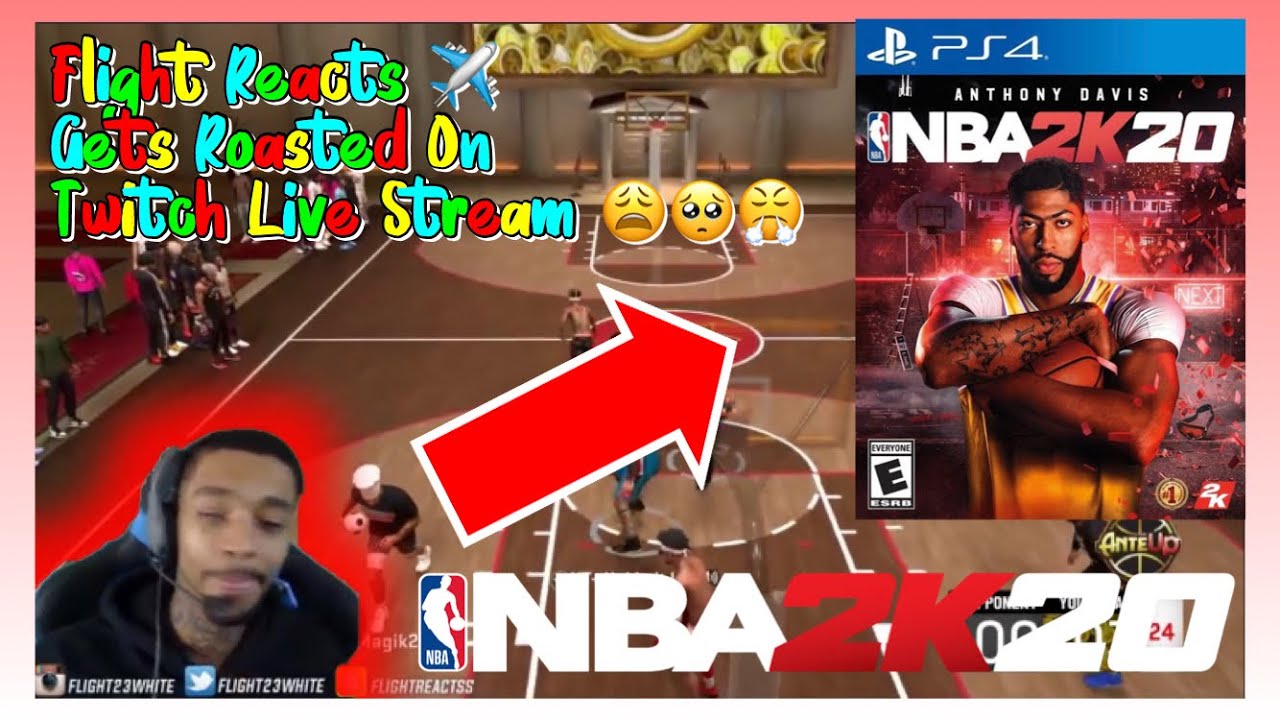### Detailed Descriptive Caption:

The screenshot depicts a vibrant image from a basketball video game, complete with a pink border adorning the left, right, and top edges of the frame. It captures a moment from a Twitch live stream where the streamer, FlightReacts, is being humorously critiqued. The top-left corner of the screen features colorful text in red, yellow, green, and blue letters reading, "FlightReacts gets roasted on Twitch live stream," accompanied by an array of emojis: an airplane, a sad face, a crying face, and an angry face. A conspicuous red arrow with a white border points emphatically towards the half-court section of the game.

On the right side of the image, the case for the game is prominently displayed. The top of the case displays the "PS4" label, while the cover features basketball star Anthony Davis wearing a yellow jersey over a white, short-sleeved t-shirt and holding a basketball against his chest. The cover also includes the "E" rating symbol at the bottom left, the "2K" logo adjacent to it, and the "NBA" logo captioned with "NBA 2K20," indicating the title of the game as "NBA 2K20."